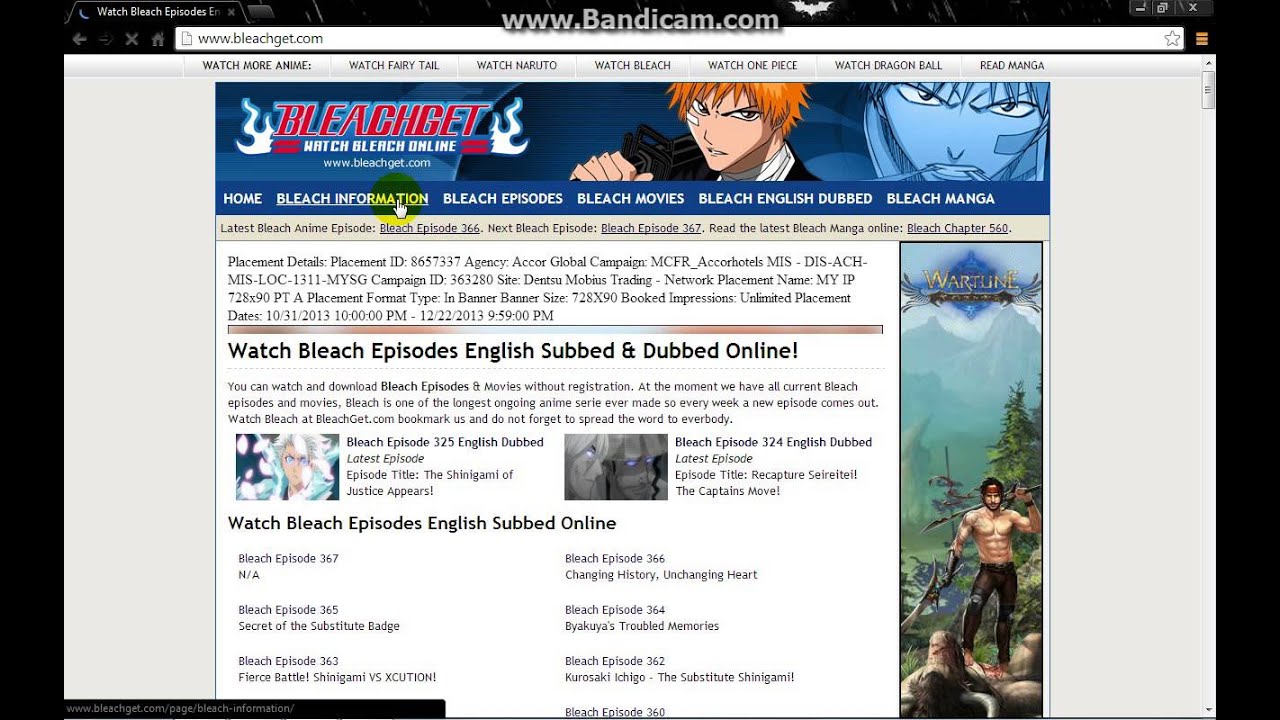The screenshot depicts a browser window featuring a website dedicated to streaming anime episodes. Dominating the top of the browser is a glossy black header with a metallic design in dark gray. In the top left corner, white text reads "Watch Bleach Episodes E," truncated by the edge of the browser tab. The tab's right side includes a dark gray "X" for closing it.

Beneath the main header, several navigational elements are visible. On the far left, a dark gray arrow is situated. Proceeding to the right, there is an expanse of negative space, followed by another dark gray "X," and a dark gray house icon. Central to this strip is the URL bar, which houses a white page icon with a gray outline and a folded top-right corner, accompanied by the URL "www.bleachget.com" in black text. At the far end of the URL bar, a dark gray star icon appears. Outside the URL field, an orange hamburger menu icon is present.

Below the black header, a light gray gradient header fades from nearly white at the top to medium gray at the bottom. This section contains tabs for navigation, separated by thin medium gray lines. The tabs are labeled in dark gray, all-capitalized text that reads, from left to right: "WATCH MORE ANIME: WATCH FAIRY TALE, WATCH NARUTO, WATCH BLEACH, WATCH ONE PIECE, WATCH DRAGON BALL, READ MANGA."

The main content of the webpage features a light gray, slightly beige-tinted column on the left and right sides, framing an image of an anime character with striking orange hair. The top right corner of the image displays red italicized, all-capitalized text: "BLEACH GET."